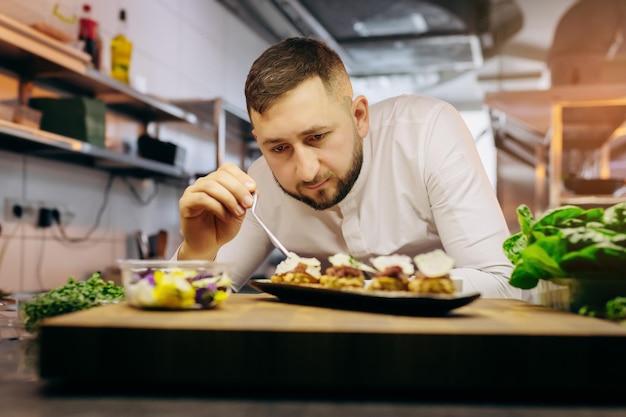In this captivating rectangular image, a focused chef with short brown hair, a full beard, and a mustache is meticulously inspecting a long, thin plate of food, possibly sushi, in a bustling kitchen setting. He is clad in a crisp white long-sleeve chef's shirt and appears to be using a silver utensil, likely a thermometer, to check the dish. The scene unfolds as if viewed from behind a wooden cutting board, adorned with a plastic cup of yellow and purple elements, possibly flowers. To the right, a bundle of fresh green leaves, possibly basil, adds a splash of color. The background reveals a well-equipped kitchen, characterized by a white brick wall, stainless steel shelves stocked with bottles, and glimpses of other silver kitchen elements, with a possible fridge and blurred outlines of additional shelves. The chef's intense concentration and the detailed kitchen ambiance highlight the intricate process of culinary artistry.